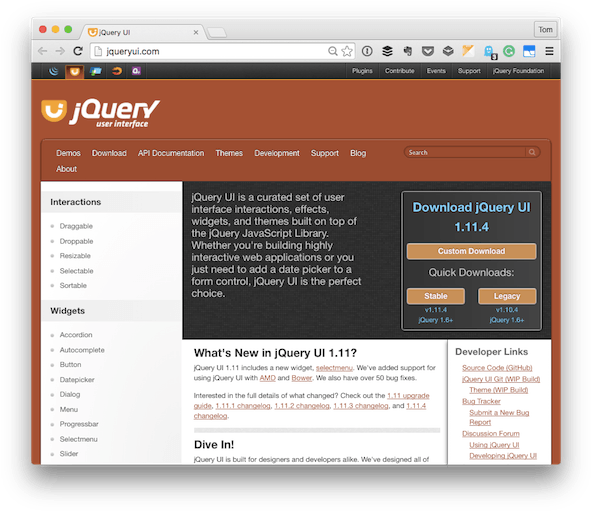The image shows an interface predominantly featuring the colors red, yellow, and green, with the words "jquery.com" appearing prominently. Various elements are arranged in a grid-like pattern with squares stacked on top of each other, some of which are marked with green checkmarks. Symbols and icons are scattered throughout the layout. Key sections include "jquery" along with terms such as plugins, contribute, event support, jQuery user interface, demos, download, pre-documentation, themes, development, support blog, ovals, search, and about.

To the left side, there is a list of interactions and widgets such as draggable, transferable, resizable, selectables, widgets recording, auto-complete, button, menu, progress bar, select menu, and author bar. Accompanying text reads: "jQuery UI has created a set of user interface interactions, effects, widgets, and themes to build and install highly interactive web applications." The layout also includes references to tools, elaborate weather units, the concept of building highly interactive web applications, and theme data.

Prominent mentions include jQuery UI downloads with versions like 1.1 and 1.4, options for quick download, stay home, legacy hosting, and support for AMD with new widgets. Overall, the image emphasizes the comprehensive offerings and functionalities of jQuery UI, encouraging users to explore and download various components to enhance their web development projects.